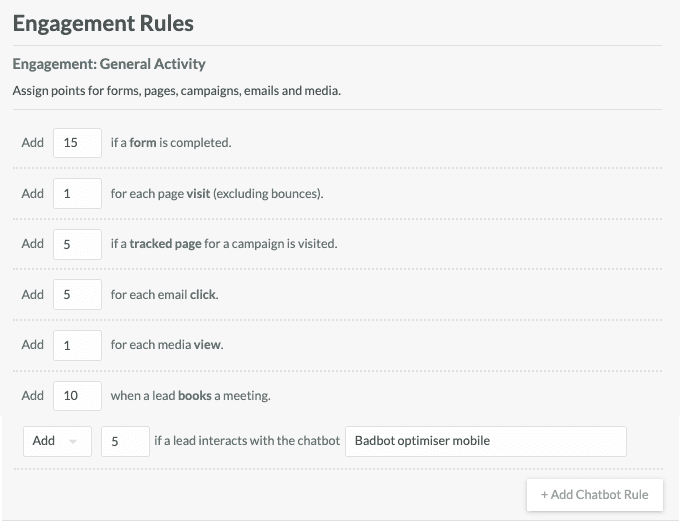This detailed image caption format consolidates all the essential points while ensuring clarity and coherence:

---

The image showcases a web page titled "Engagement Rules," which outlines a point-based system for measuring user engagement within a tech context. The rules specify different activities and their corresponding point values, such as the assignment of 15 points for form completions, 1 point for each page visit (excluding bounces), 5 points for visiting a tracked page or campaign, 5 points for email clicks, 1 point for media views, 10 points for booking a meeting, and 5 points for interacting with a chatbot. The chatbot rule configuration is denoted as "Bad Bot Optimizer Mobile." The system appears to be flexible, allowing users to modify point values based on their preferences to suit their specific engagement measurement needs. At the end of the page, there is an "Add Chatbot Rule" button that offers additional customization options.

---